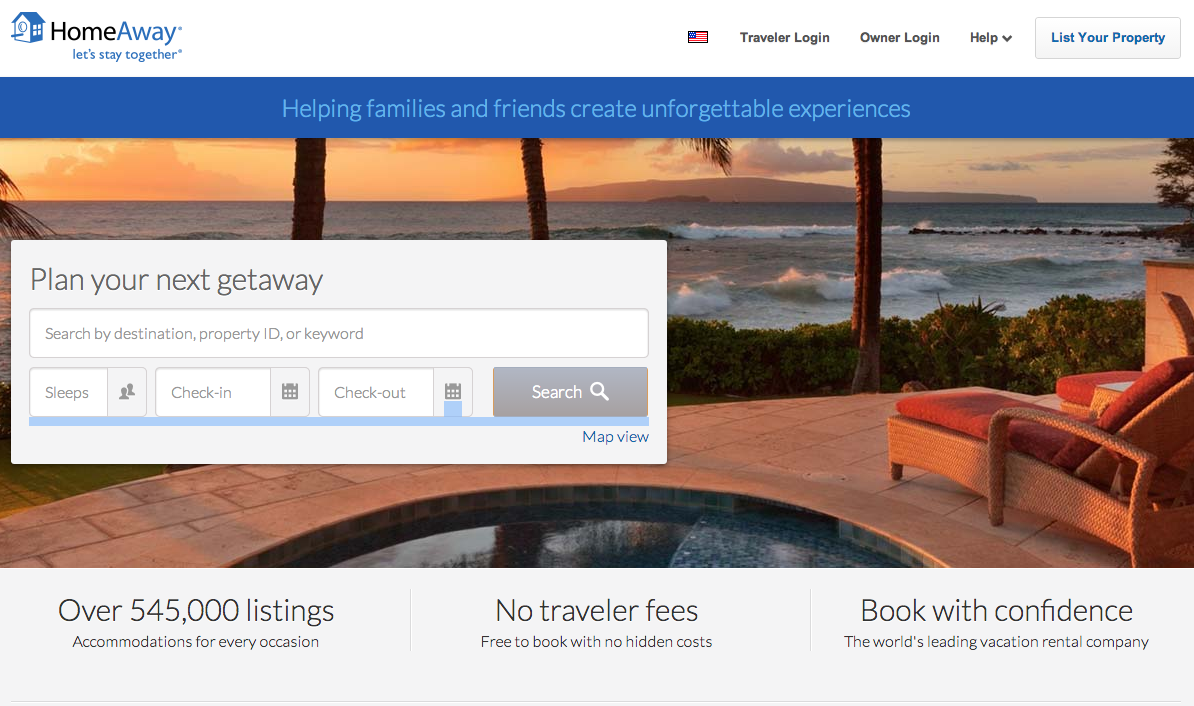This image depicts the homepage of the HomeAway website. Dominating the top section is the HomeAway logo, accompanied by the tagline "Let's Stay Together" and a small blue house icon. The navigation menu includes sections such as "Traveler Login," "Owner Login," and "Help." 

Prominently featured in blue is a button encouraging users to "List Your Property." A striking blue banner stretches across the homepage, proclaiming, "Helping Families and Friends Create Unforgettable Experiences." Beneath this banner, users are invited to plan their next getaway with a search function that allows for searches by destination, property ID, or keyword. 

Additional search options include selecting the number of guests ("Sleeps"), check-in and check-out dates, each with associated calendar icons, and a search field accompanied by a small magnifying glass icon. A "Map View" button is also available. 

Key selling points of the site are highlighted, including "Over 545,000 Listings," "Accommodations for Every Occasion," "No Traveler's Fees," "Free to Book with No Hidden Costs," and "Book with Confidence" as it is described as the world's leading vacation rental company. 

The background of this webpage features a picturesque ocean property at sunset, showcasing a small pool area, lounge chairs, and an abundance of lush trees.